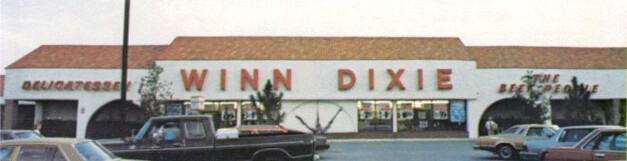The image depicts a long white building with a striking red roof, featuring a central section that is noticeably taller and longer than the flanking wings. Dominating the front of this central section are bold red letters spelling out "WINN-DIXIE." To the left side of the building, a sign in matching red letters reads "Delicatessen." The right side of the building showcases archways with signage hinting at "Bee People," using "Bee" with two Es, evoking the imagery of honey bees. Several cars are parked in front, suggesting a spacious parking area. The wide entrance beneath the central portion of the building appears to serve as an access point, possibly for a fuel station.